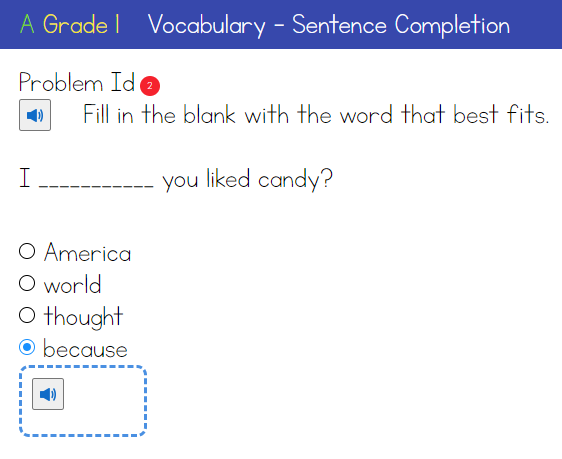This image is a screenshot from a grade one educational lesson, accessible via a computer or an app. At the top of the screen, there is a banner with a gradient of purplish blue. Within this banner, large green letters spell out "A, A," followed by "Grade One" in bright yellow text. Underneath, in white text, it reads "Vocabulary - Sentence Completion."

Below the banner, on a white background, the text starts with "Problem ID," next to which is a red circle containing the number "2." Accompanying this is a small audio icon. The instruction "Fill in the blank with the word that best fits:" appears next, guiding the user through the task. The sentence to be completed reads, "I ..... you liked candy?" with several dots symbolizing the blank space to be filled.

Directly beneath the sentence, there are four answer options, each accompanied by a circle that can be selected:
1. America
2. World
3. Thought
4. Because

The circle next to the word "Because" is highlighted in blue, indicating it is the selected option. Below these options, there is another audio icon encased in a blue-rectangle border, emphasizing its interactive functionality.